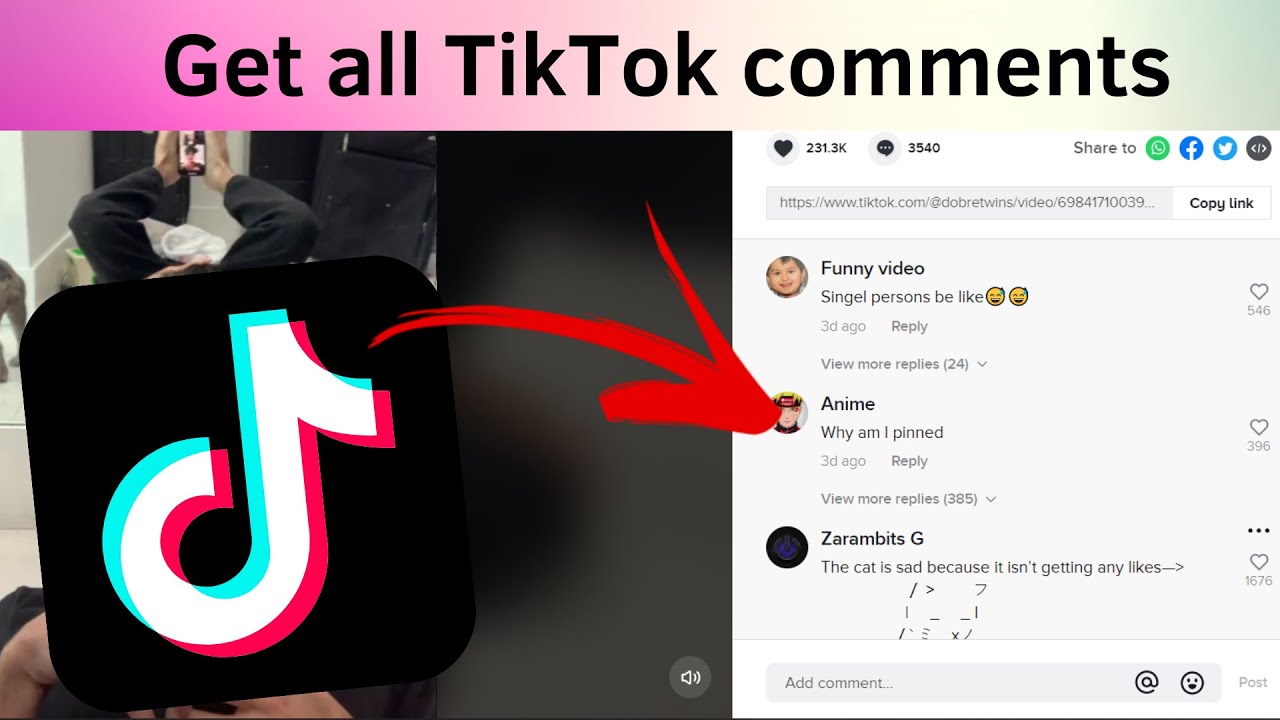The image is a combination of a screenshot and a meme creation. At the top, a multicolored box contains the text "get all TikTok comments" in black font. On the left side of the image, there's a picture showing someone's feet holding their phone, with a person's arms visible near the bottom. The TikTok logo is prominently overlaid on top, obscuring some details of the individual in the picture. From the TikTok symbol, a red arrow points toward a screenshot of comments.

In the screenshot, the top left corner displays 31.3K hearts and 3,540 comments. To the right, there are sharing options for WhatsApp, Facebook, Twitter, and an unfamiliar icon, alongside a link and a "copy link" button.

The first comment shown is from a user named "funny video," with a profile picture of a small child, who wrote, "single persons be like," followed by several laughing emojis. Below this, a user named "anime" asks, "why am I pinned?" with an arrow pointing to their profile picture, which the red arrow highlights. The final comment is from "Zarin Bitschi," stating, "The cat is sad because it isn't getting any likes," accompanied by an arrow pointing to the right.